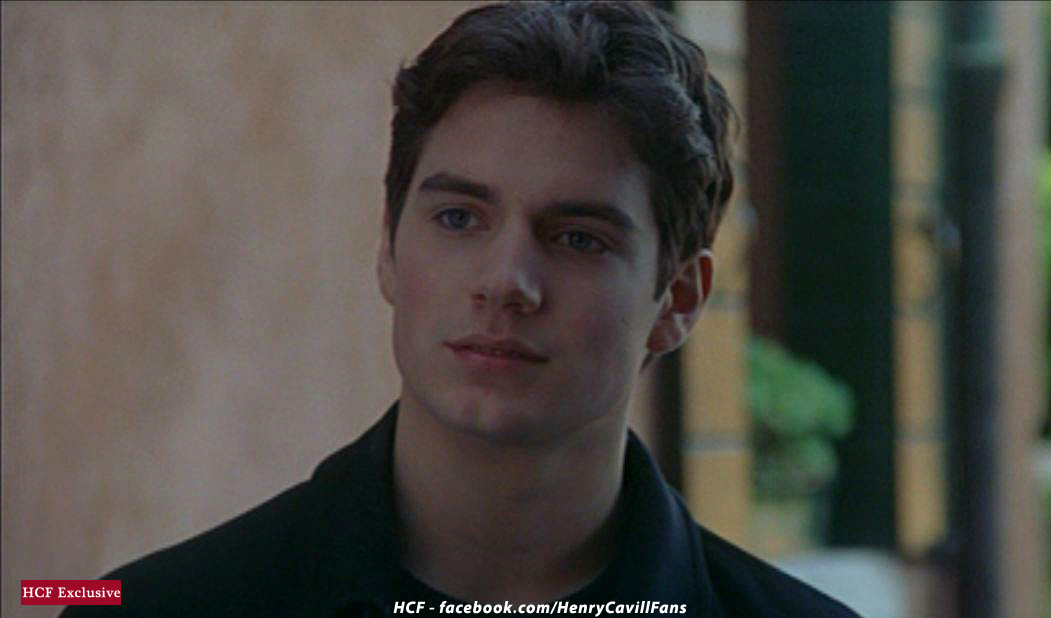This close-up photograph captures a young man, potentially in his late teens to early twenties, who strongly resembles Henry Cavill. He is looking slightly to the left of the camera while maintaining a neutral, pleasant smile. His thick brown hair is styled fashionably short, complementing his blue eyes, well-defined chin, and thick eyebrows. He is wearing a dark blue or black collared shirt, which could possibly be paired with a darker jacket.

The background is blurred, but details suggest a mix of an indoor and outdoor setting. To the left side of the image is a light tannish wall, while the right side reveals an outdoor environment that appears sunny with some green plants. At the bottom left corner of the image, there is a red rectangular strip containing white text that reads "HCF EXCLUSIVE". Additionally, at the very bottom center in white text, it says "HCF - facebook.com/HenryCavillFans".